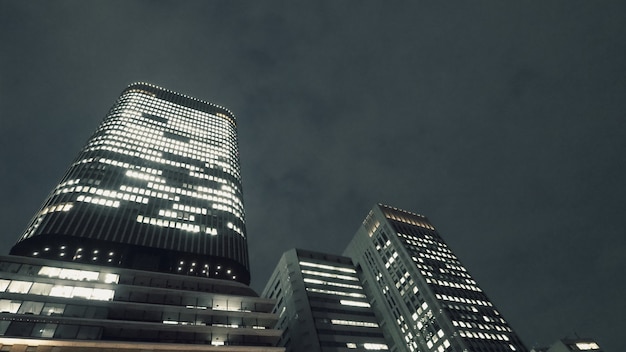This black-and-white nighttime photograph captures a dramatic upward angle shot of towering office buildings against a sky mottled with dark and light gray clouds. Dominating the scene to the left is a particularly tall and wide building with the majority of its office lights on, though patches of darkness indicate some lights are off. This building appears to ascend sharply, almost as if it's shooting into the sky, a perspective further emphasized by its angle. Below or perhaps behind it, another prominent building emerges, smaller and darker in tone but equally illuminated by an array of lights. On the right, yet another high-rise stands tall with most of its windows aglow. The buildings generally have a rectangular shape and extend impressively high, though the specific visibility of their corners varies due to the angled perspective. In the bottom-right corner, a shorter building is discernible, possibly farther in the distance, with blurry, illuminated lettering that's difficult to read distinctly. The overall composition creates a striking contrast between the illuminated buildings and the brooding night sky, accentuating the architectural grandeur of the cityscape.